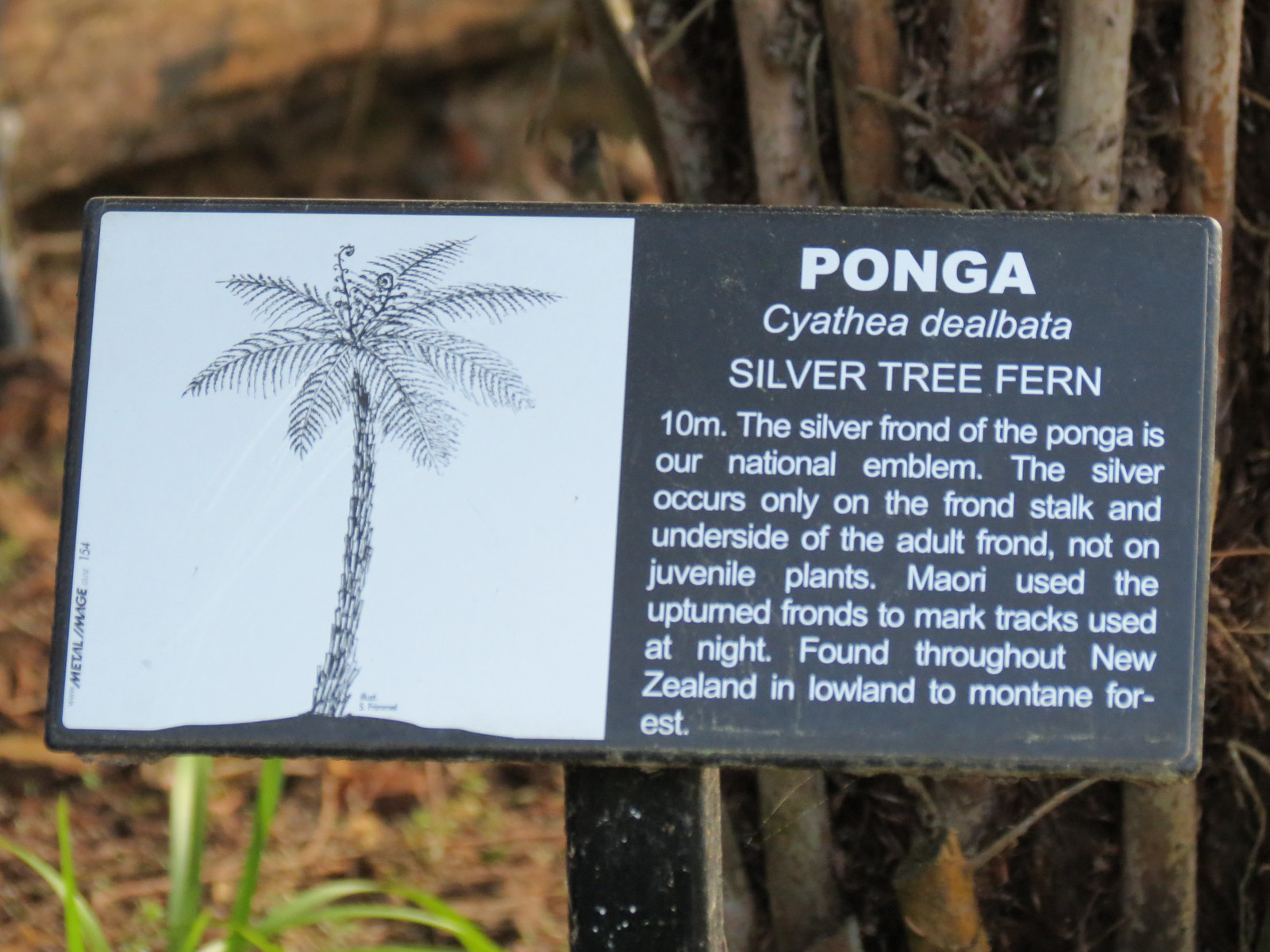The photograph captures an informational plaque securely attached to a squared single pole, both painted black. The left half of the black plaque features a detailed black-and-white drawing of a tall palm-like tree with fronds, identified as the Ponga, also known as the Silver Tree Fern. On the right half, against the black background, white text provides detailed information: "Ponga, Cyathea dealbata, Silver Tree Fern, 10 meters." It notes that the silver frond of the Ponga is New Zealand's national emblem. This distinctive silver hue only appears on the frond stalk and underside of the adult frond, not on juvenile plants. Maori people use the upturned fronds to mark trails used at night. The Ponga is found throughout New Zealand, from lowland to montane forests. The foliage in the background of the image is slightly out of focus but complements the plaque's detailed description of this iconic plant.